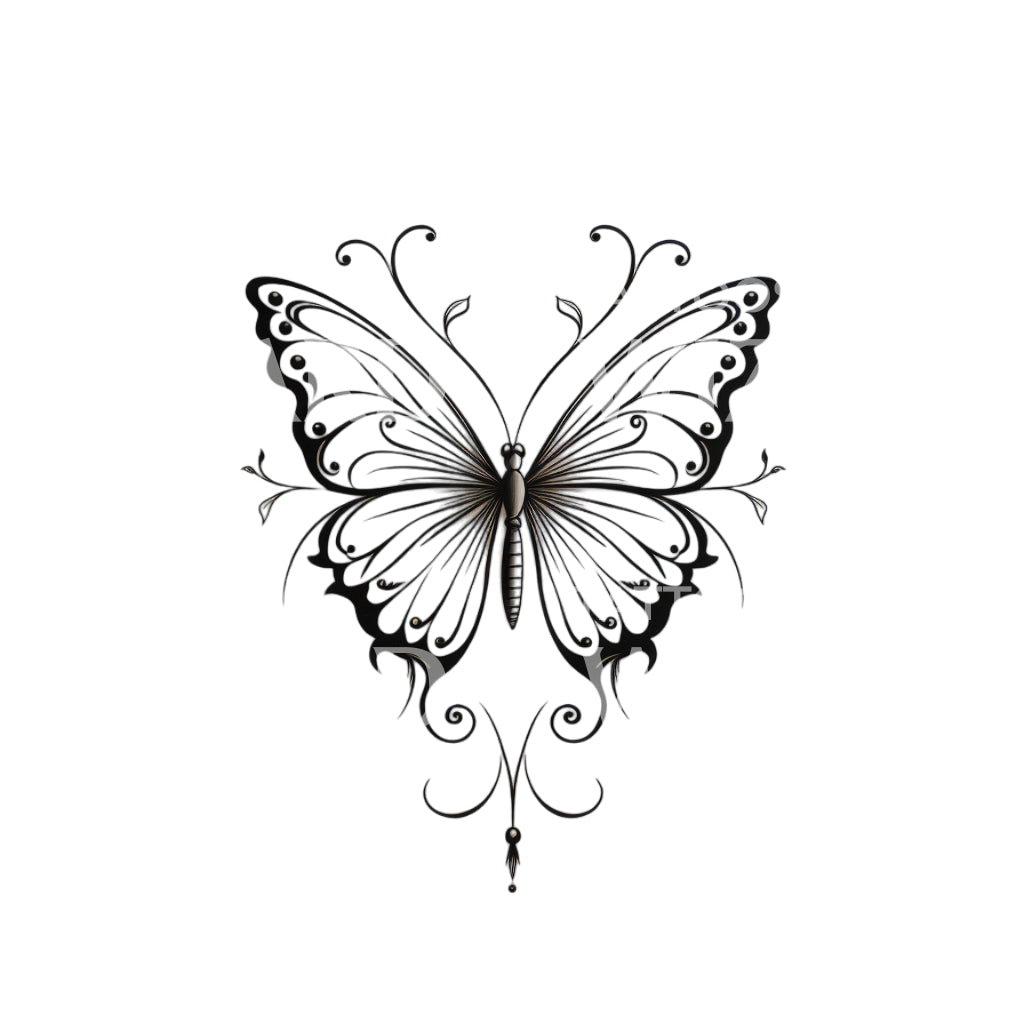This is an elegant, stylized black and white ink drawing of a butterfly viewed from above. The butterfly's body is centrally positioned with very long antennae that extend upwards, ending in elaborate curls. The wings feature dark black edges and are adorned with black dots and curved lines indicating striations. Decorative curls and thin spindly extensions, some resembling leaves, extend from the center and bottom edges of the wings, enhancing the fantastical appearance of the illustration. There is also a small humanoid figure below the butterfly, adding to the whimsy of the piece. The overall composition is richly detailed and symmetrical, making it an eye-catching piece of art.